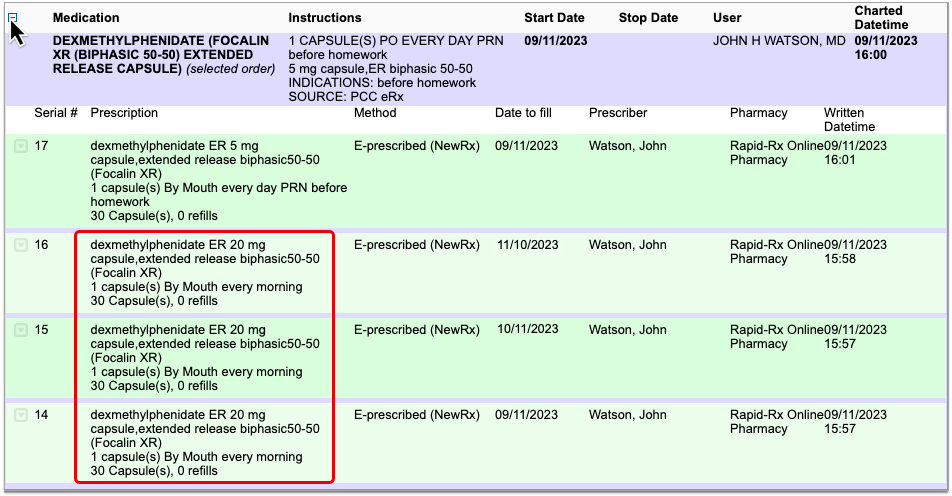This image depicts a color-coded spreadsheet displayed on a website. The spreadsheet is organized with columns and rows, featuring varying shades of purple and green for easier readability. The top row is highlighted in purple, immediately followed by a green row. This pattern continues with a thin purple line separating each subsequent green row. Notably, the first and third green rows are in a darker shade compared to the second and fourth green rows.

The header, formatted in purple, labels each column as follows: "Medication," "Instructions," "Start Date," "Stop Date," "User," and "Charted Date Time." The list of medications includes complex names such as dimethylene and folcaline, indicating prescriptions managed carefully. 

Each row is completed with corresponding dates and details, signifying the organized schedule of medication administration. The entire chart is attributed to prescriber John Watson.